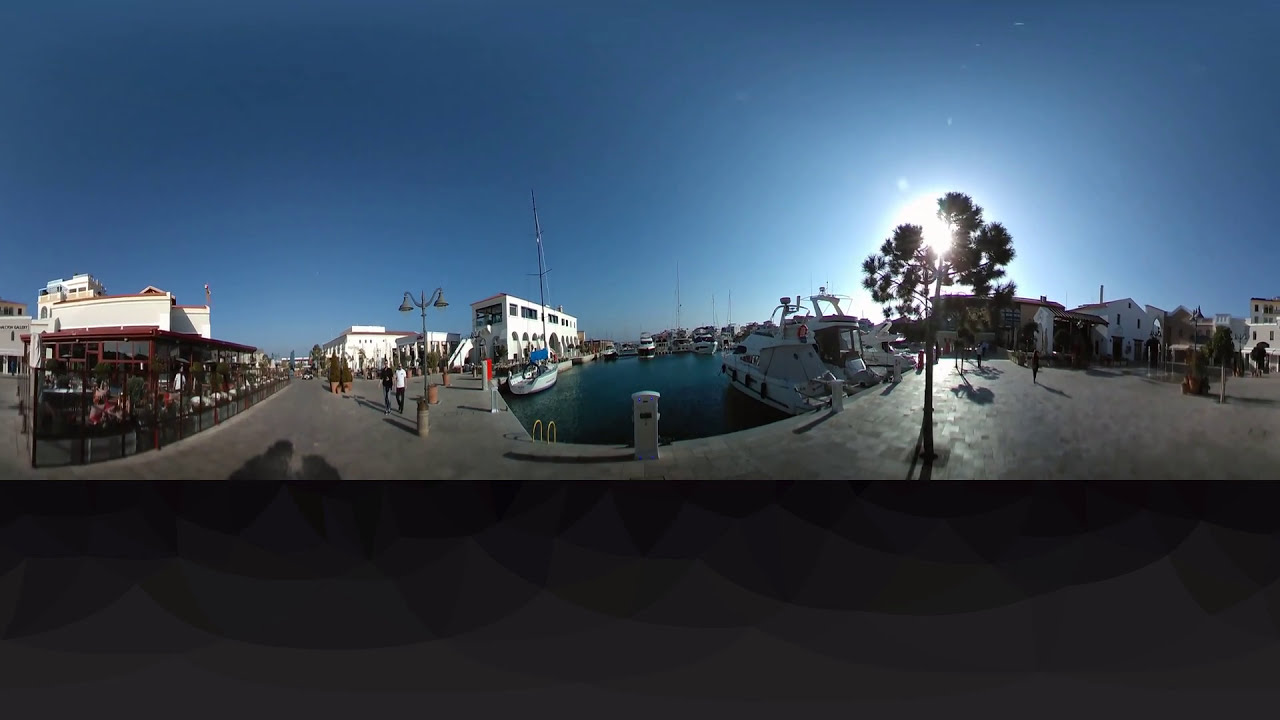This image captures a twilight scene in a bustling commercial area, shot with noticeable distortion. The sky is a deep dark blue, indicative of the time just after sunset. The horizontal rectangular frame features a large dark border along the bottom, anchoring the visual elements.

On the left side of the image, white buildings, possibly part of an arcade or outdoor entertainment area, stand backlit by the dwindling sunlight. People are seen walking away from the camera along a dark gray street, possibly heading towards a tourist attraction or a wharf. These buildings gradually transition into what looks like a more distant cluster of buildings or houses. A tree, seemingly growing in the middle of the street, adds an interesting focal point and further emphasizes the image's distortion and bending angles.

To the right, the scene extends towards what appears to be a wharf or pier, with boats docked and a possible entrance to the water. The presence of a setting sun behind a tree on this side creates a dramatic interplay of light and shadow, casting an enchanting glow over the entire area. The overall composition suggests a mix of urban and natural elements, blending the dynamic human activity with serene waterfront tranquility.